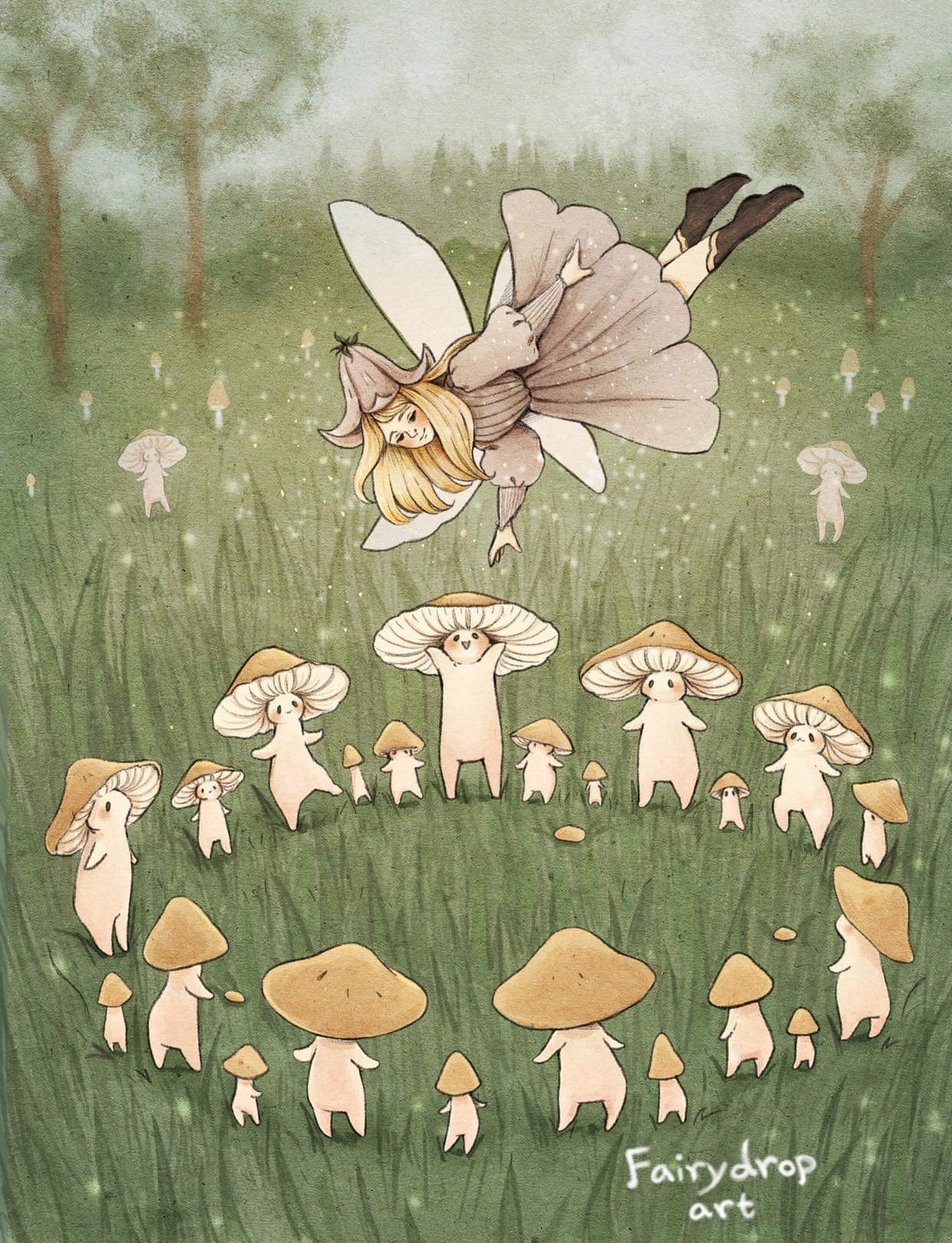This detailed painting captures a whimsical fairy ascending gracefully above a circle of anthropomorphic mushrooms on a lush green grassy ground. The enchanting fairy, depicted with long blonde hair, is adorned with a delicate flower hat and wears a long-sleeve pink dress that reaches her knees. Her white wings shimmer as she hovers, feet pointed towards the top right of the image, while her face is turned towards the bottom center with a gentle smile. The fairy's look is completed with black boots. In the foreground, a ring of mushroom people, characterized by their light brown caps, human-like faces, arms, legs, and feet, eagerly gaze upwards at the fairy. These mushroom beings create a playful and magical scene as they extend their small arms towards the enchanted fairy. Additional mushroom figures and trees surround the scene, adding depth and richness to the landscape. In the bottom right corner, a handwritten text reads "fairy drop art," anchoring the charming narrative within the painting.